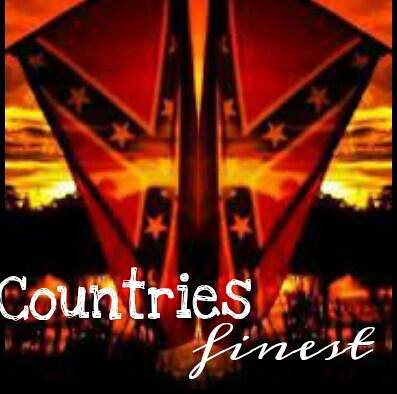In the image, there is prominently displayed text reading "Country's Finest." The background is dominated by a stunning sunset, casting vibrant hues of red and orange across the sky. The sun itself is partially visible, peeking out from behind a cluster of trees. This picturesque sunset serves as a backdrop for what appears to be a flag or possibly two flags side-by-side. The flag has distinctive red coloring, accompanied by blue and white stripes, and white stars set against blue. Its unique shape is somewhat reminiscent of a Confederate flag, though its exact nature is ambiguous, adding an element of intrigue. The flag's configuration and its almost upside-down triangular form also suggest it could alternatively be a kite.